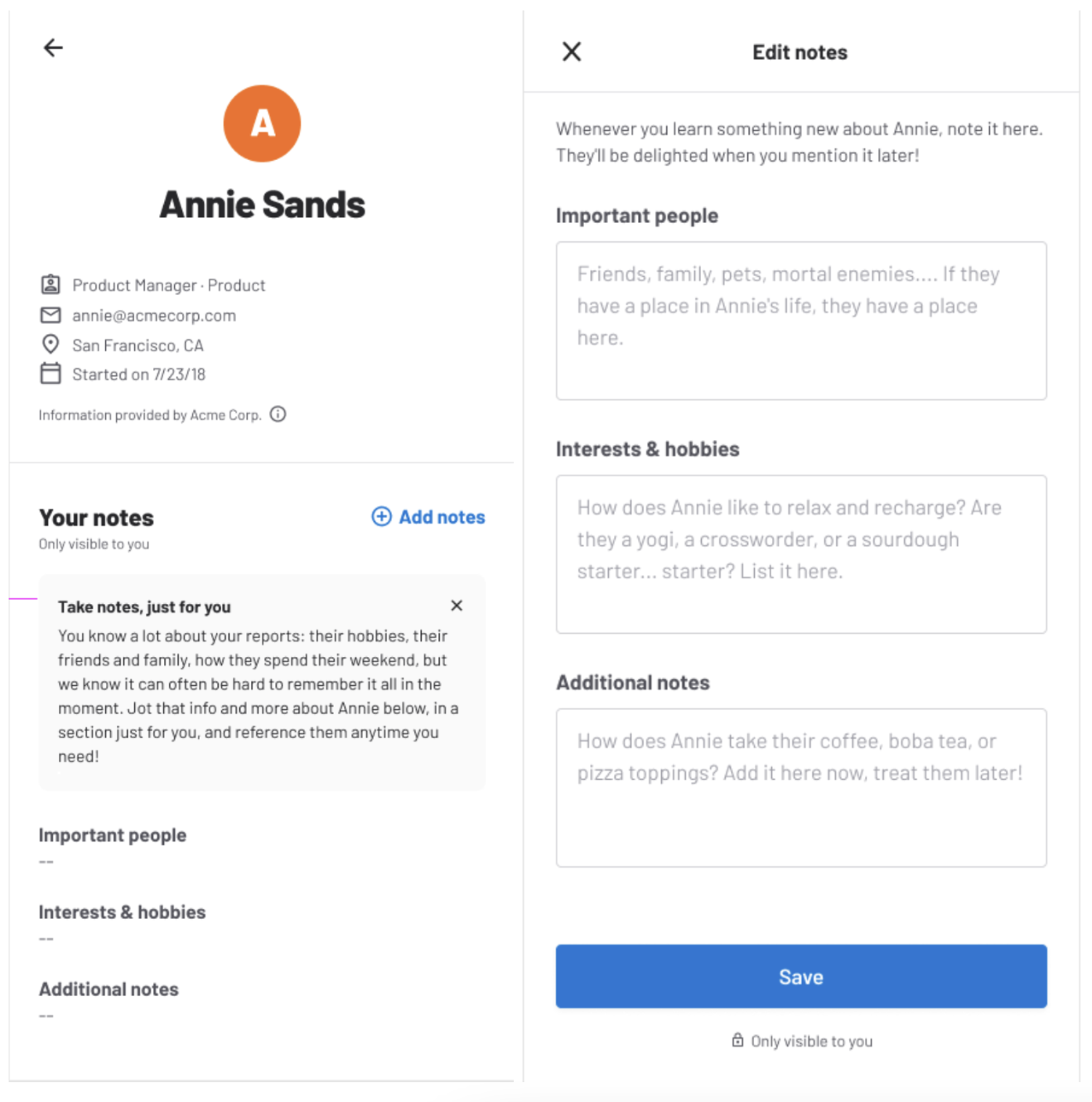**Detailed Caption:**

This composite image consists of two mobile screenshots displayed side by side, tightly cropped to focus on the content without revealing the browser or operating system.

**Left Screenshot:**
- The left side of the image features a user profile summary. A black arrow is pointing left, guiding the user towards potential navigation.
- At the top, there is an orange circle containing a white letter "A," representing the first initial of the user's name. Below the circle, the name "Annie Sands" is displayed in bold, black text.
- The profile further details:
  - Job Title: **Product Manager, Product**
  - Email: **Annie@AcmeCorp.com** (preceded by an envelope icon)
  - Location: **San Francisco, California** (preceded by a locator map icon)
  - Tenure: **Started on July 23rd, 2018** (preceded by a calendar icon)
  - Source: **Information provided by AcmeCorp** (with an info icon for additional details)
  
Below the profile details, there's a section labeled "Your Notes," presented largely in black text with the phrase "only visible to you" in smaller, bolded print. There is a blue plus icon to add more notes accompanied by the text "take notes just for you."

A descriptive paragraph encourages users to jot down personal information about Annie, such as hobbies, friends, family, and weekend activities. This section aims to help the user remember essential details for future reference. Additional expandable categories include "Important People," "Interests and Hobbies," and "Additional Notes."

**Right Screenshot:**
- The right half presents an interface titled "Edit Notes" with an "X" button to close the editor.
- The top section prompts users to jot down new information about Annie, suggesting that recalling and mentioning these notes later will be appreciated by her.
  
It includes the following expandable categories:
  - **Important People:** A placeholder text like "friends, family, pets, mortal enemies" suggests listing significant individuals in Annie's life.
  - **Interests and Hobbies:** Users are encouraged to record details about how Annie likes to relax, with examples such as yoga, crossword puzzles, and sourdough baking.
  - **Additional Notes:** Prompts for specific preferences like coffee types, boba tea flavors, and pizza toppings, with a note to record now and treat the person later.

Overall, the dual screenshots illustrate a sophisticated app designed to help users keep track of detailed personal and professional information about their contacts, potentially enhancing both professional relationships and personal rapport.